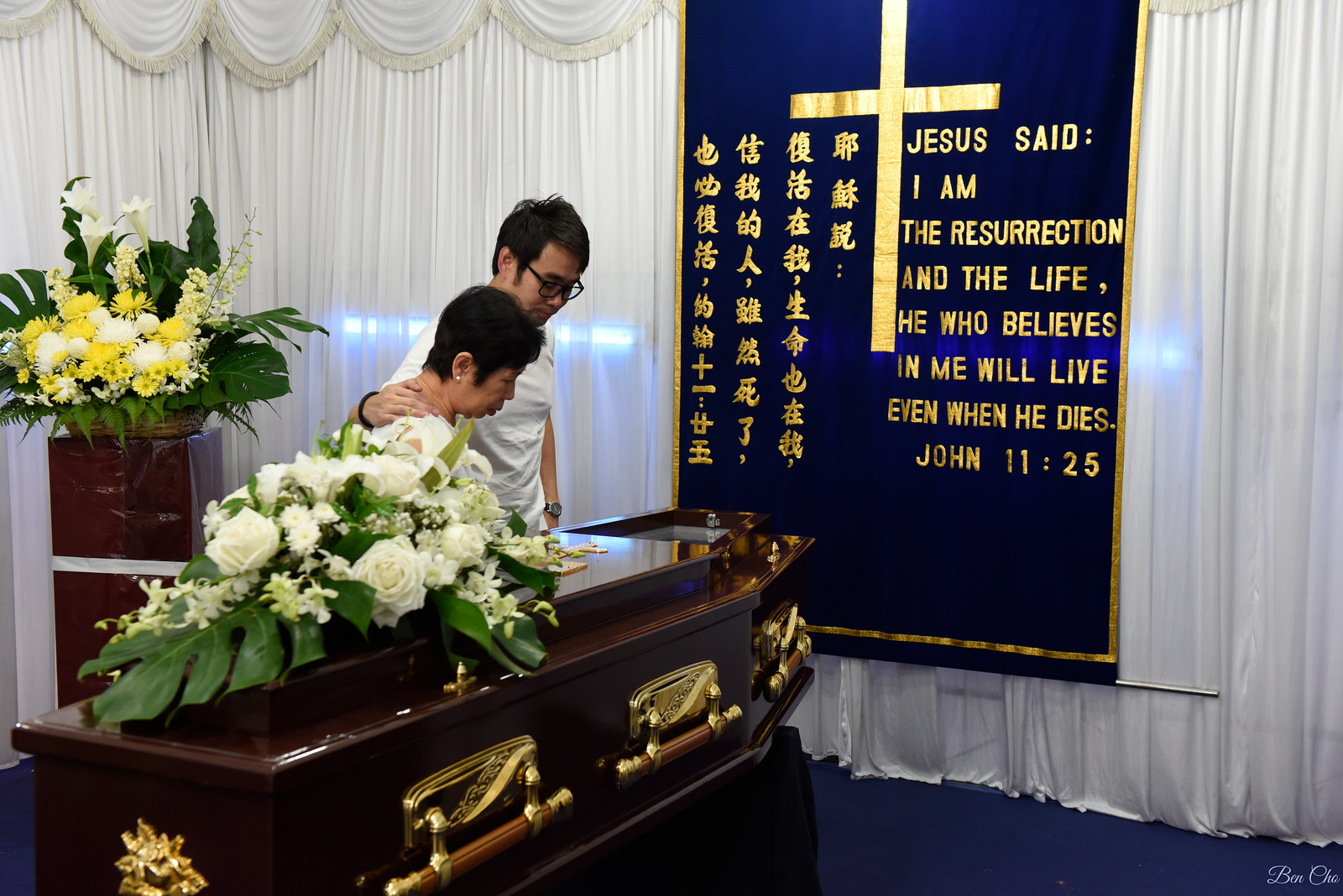The image captures a solemn funeral scene set indoors, likely in a funeral home. The room is draped with white curtains, covering the windows and creating a somber atmosphere. Prominently featured in the lower left quadrant of the image is a shiny brown wooden coffin adorned with gold handles and gold accents. Atop the coffin rests a bouquet of white roses and other various white flowers, interspersed with greenery.

Standing at the head of the coffin are two individuals, a man and a woman, both appearing to be of East Asian descent and dressed in white shirts. The man, who wears glasses, has his right arm gently around the woman, who is adorned with white earrings. Both have sorrowful expressions as they gaze down at the coffin. 

In the background, situated behind the couple and the coffin, is a large floral arrangement of yellow and white flowers with greenery. Additionally, on the left side of the image, there appears to be a pillar or file cabinet topped with another flower arrangement of similar colors.

Hanging on the right side of the image against the white drapes is a blue banner featuring a gold cross and four columns of oriental characters. Alongside these, it bears an inscription in gold lettering that reads, "Jesus said, I am the resurrection and the life. He who believes in me will live, even when he dies." (John 11:25). The floor beneath them appears to be a navy carpet, completing the dignified setting.